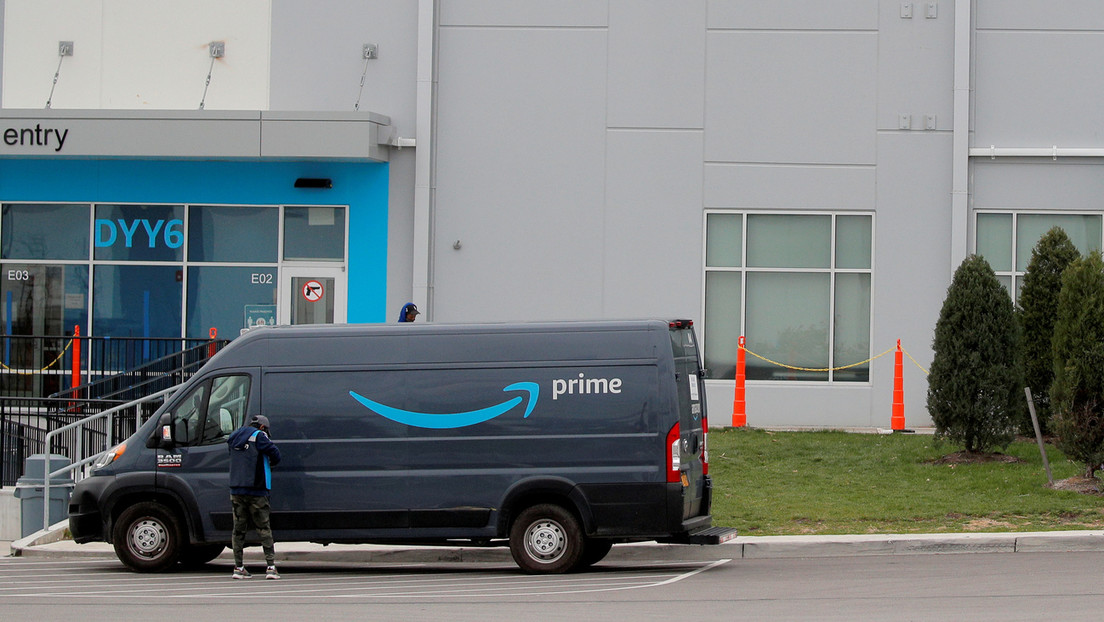A photograph captures an Amazon Prime delivery van and its driver, poised at the door, ready to begin their route. The driver is wearing a dark navy windbreaker or rain jacket, a ball cap, camouflage leggings, and tennis shoes, exuding practicality and readiness for any weather conditions. The long delivery van is painted in navy blue, adorned with a light blue arrow and the word "Prime" prominently on its side. The backdrop features a concrete building in muted gray and white tones, accented by blue-painted window frames. The setting appears to be an Amazon facility, as suggested by the light blue stenciling on one of the windows, which displays "DYY6" in capital letters and the word "entry" under a small awning at the door. The driver seems either to have just completed a delivery or is preparing to embark on a new one, capturing a moment of everyday efficiency in the logistics chain.